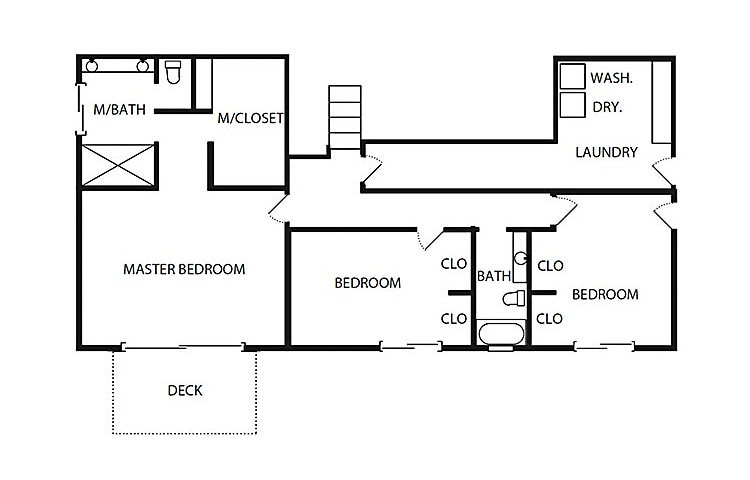This black and white blueprint image, set against a white background with no visible borders, details the layout of a three-bedroom, two-bathroom house. Upon entering from the staircase located centrally, to the left is a hallway leading to the laundry room, clearly marked with positions for a washer and dryer, and an exit door to the outside. 

To the right of the stairs lies the entrance to the master suite. This suite features a spacious master bedroom with a sliding glass door that opens onto a deck, outlined with a dotted rectangle. Adjacent to the master bedroom is a hallway that splits; to the left, it leads to the master bathroom equipped with two sinks, a toilet, and a combined tub-shower, while to the right, it leads to the master closet.

Further right in the floor plan, past the master suite and through another hallway, you encounter two additional bedrooms, each with two closets. Nestled between these bedrooms is a shared bathroom. Notably, there are doors in both the second and third bedrooms leading outside, although no additional decks are specified. The visualization is completed by the stairs that likely provide access to another level, either above or below the depicted floor.